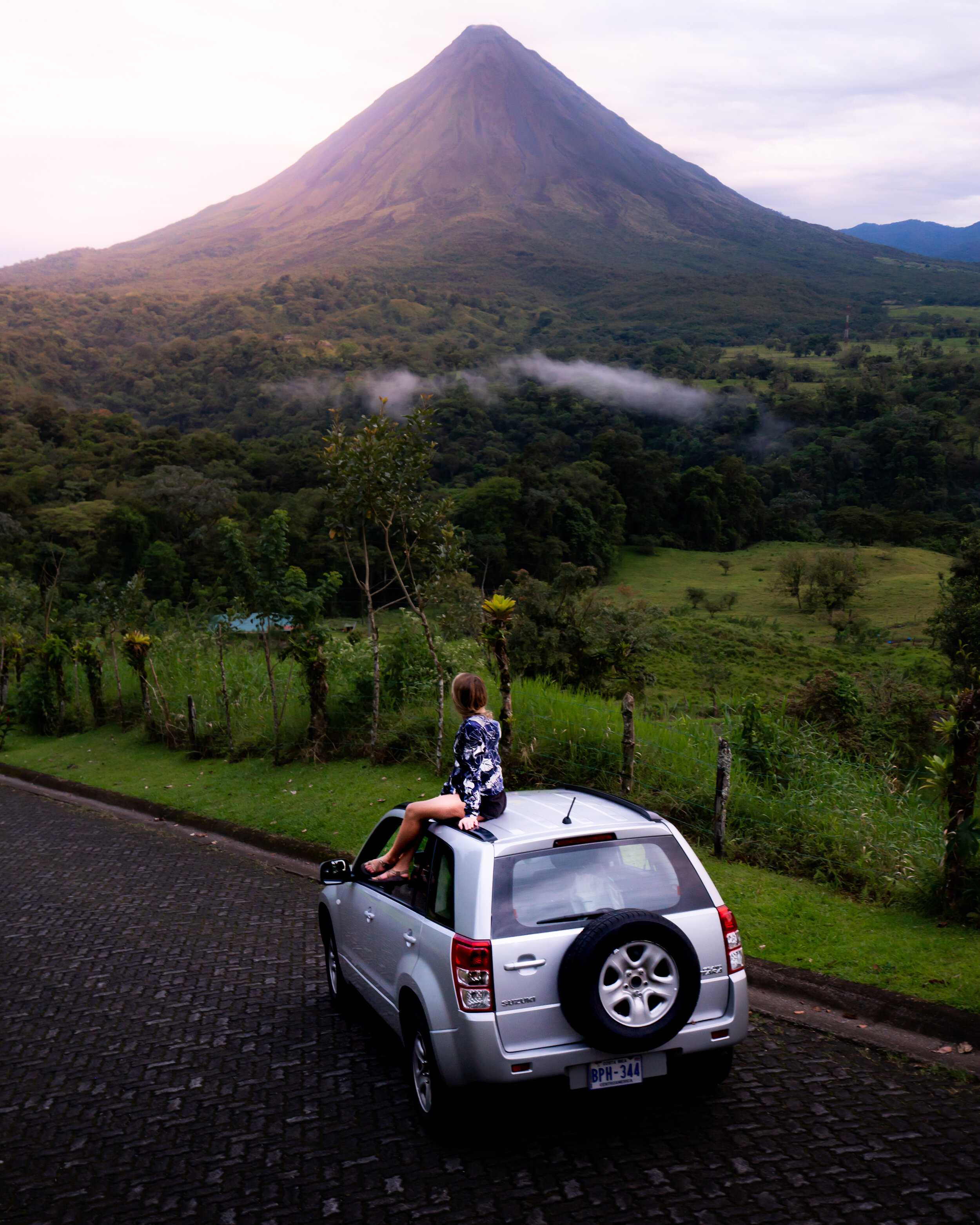This photograph captures a serene landscape featuring a dormant volcano in the background. The volcano, brown at the summit, transitions into lush green vegetation as it descends, with a dense forest of trees stretching across the entire width of the image. A small, fluffy cloud hangs in the sky above the treetops. In the midground, the forest gives way to a grassy field with a scattering of trees and a rustic fence adorned with flowers and wooden posts. In the foreground, a silver car is parked on a road that runs from the middle left to the bottom right corner of the image. Seated on the roof of the car is a woman, gazing out at the breathtaking scene. The palette of the image includes blues, whites, blacks, browns, grays, greens, and yellows, but no text is visible. This idyllic scene beautifully captures the peaceful coexistence of human presence and natural splendor.